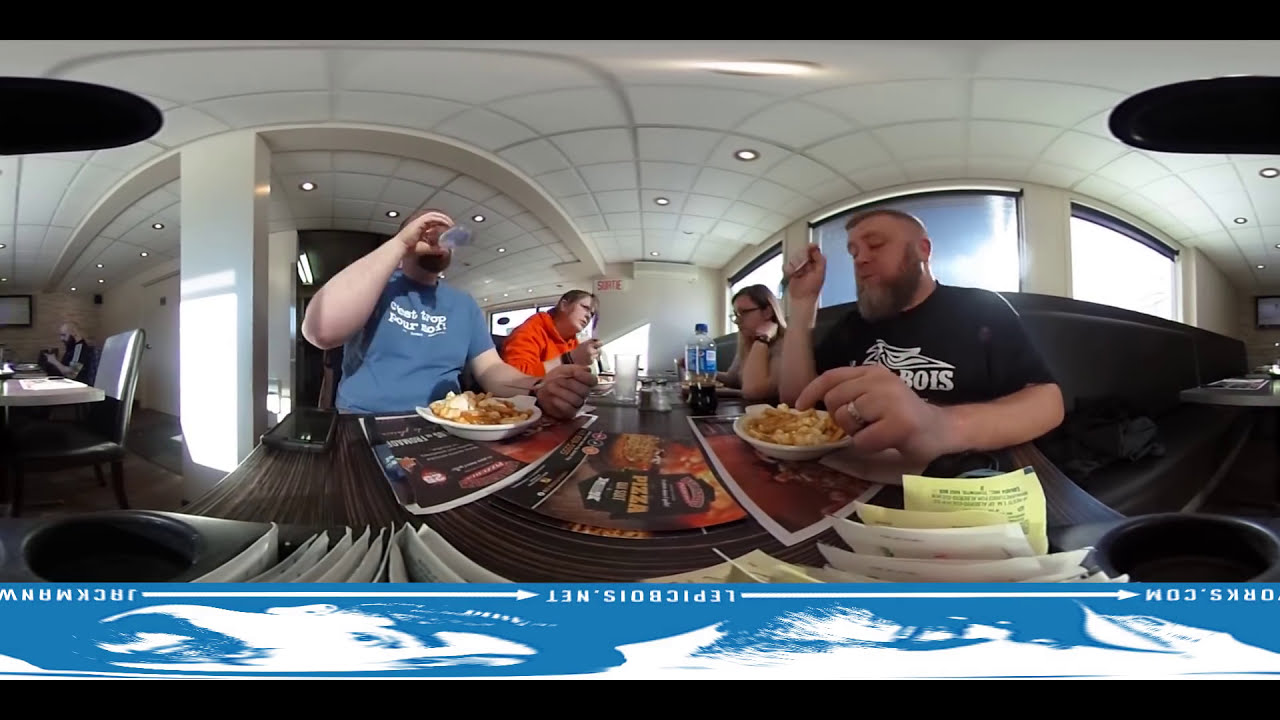In this image, taken with a fisheye lens that distorts the dimensions, we see four people - two men and two women - sitting around a dark wooden table in a restaurant with white walls and a grid-style ceiling. The setting, likely a pizza restaurant due to a visible placemat advertisement for pizza, features brown hardwood floors and possibly some carpeting. The group is actively eating and drinking; one man with a beard, wearing a black shirt, is eating mac and cheese, while another is drinking from a raised glass. A woman sitting next to the bearded man wears a watch and appears to be engaged in conversation with the woman across from her, who is dressed in a bright orange shirt. The man across is in a blue shirt with text on it, and there’s a Diet Coke bottle on the table near him. The table also holds a variety of items including menus, salt and pepper shakers, sugar packets, cups, and possibly brochures or advertisements. Additional recessed lighting lends to the overhead illumination, while in the distance, more tables with other diners and windows can be seen, indicating it’s daytime. The composition and colors in the image include black, white, yellow, tan, blue, and orange, with the main focus being on the central group of people enjoying their meal amongst a bustling, brightly lit indoor restaurant atmosphere.